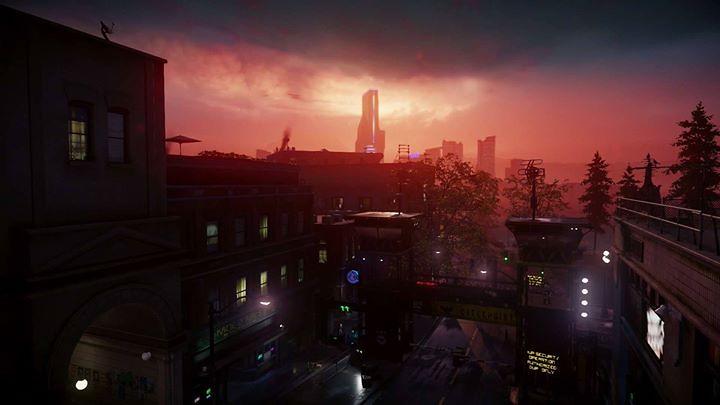This photograph captures an evocative scene that resembles concept artwork from a movie or video game. Taken during the late hours of the day, the image is characterized by a stark contrast between its darkened foreground and the vivid, red-hued sky in the background. The dimly lit street in the foreground is illuminated by glowing streetlights and features a small bridge crossing over it. To the left side of the street, two shadowy buildings, likely apartment complexes, add an urban texture, though their details are obscured by the encroaching darkness.

Further into the distance, additional buildings populate the scene, with one notably tall structure piercing upward and silhouetted against the fiery sky. This striking sky features a gradient of bright red, punctuated by patches of luminous clouds at its center, and fades to a darker tone as it ascends, suggesting an intense celestial event or possibly something otherworldly descending from space. The juxtaposition of the illuminated street and the dramatic sky creates an atmosphere of anticipation and otherworldly beauty.